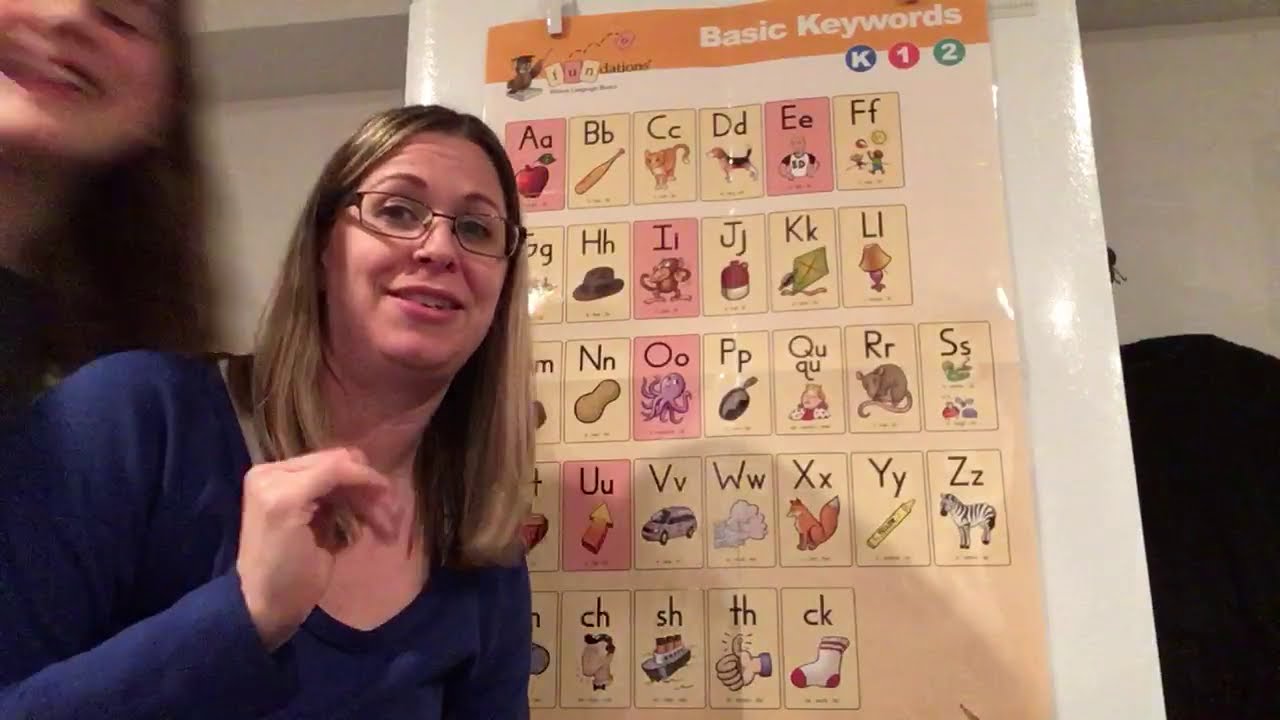In the foreground of this horizontal, rectangular image, a Caucasian woman is slightly turned towards the right, her body facing roughly the five o'clock position. She has shoulder-length, straight blondish-brown hair, and is wearing wire-rimmed black glasses along with a long-sleeve, V-neck blue shirt. She appears to be in her 20s and is making a 'C' shape with her right hand, which is raised to her chest level. Her mouth is open, capturing a slightly surprised but positive expression.

In the upper left corner of the image, a blurry but smiling young woman with long brown hair can be seen. The blur suggests she's in motion. Both women are in what looks like a classroom setting.

Behind them, there is a large beige-colored board featuring a white-bordered poster. The poster is titled "Basic Keywords" with "K1 and 2" encircled beneath the title. The poster displays the entire alphabet with each letter shown in both uppercase and lowercase. Each letter is accompanied by an illustration: for example, 'A' is paired with an apple, 'B' with a bat, 'C' with a cat, and so forth. The letters and images are presented in rectangular backgrounds, providing a clear and educational visual aid.